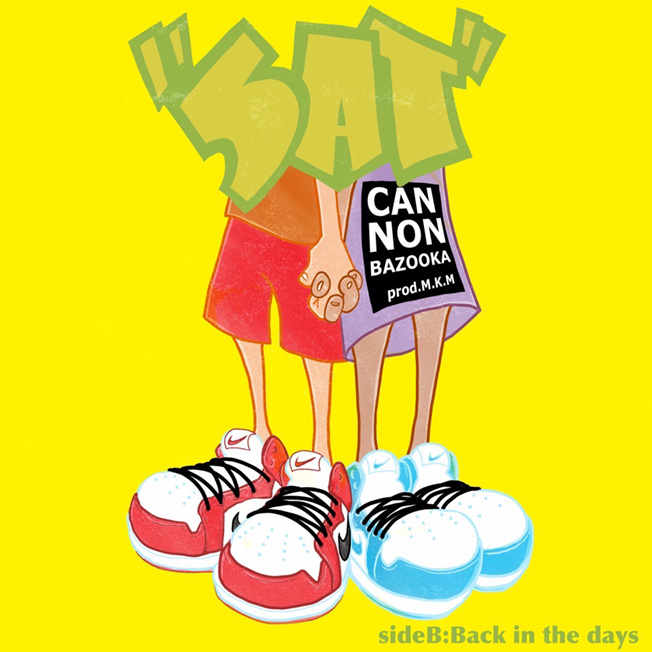The animated image appears to be a stylized, urban graffiti-inspired design, potentially serving as the cover for an EP or record. Dominating the scene are two human figures, one lighter-skinned wearing an orange shirt and red shorts, and the other darker-skinned in a purple dress. They are holding hands. Both figures sport exaggerated Nike sneakers—one in red and white, the other in blue and white—all with black laces. At the top, the text "SAT" or "5AT" is prominently displayed in graffiti-style green lettering with quotation marks. The purple dress features a black square containing white text that reads "Cannon Bazooka PROD. MKM." At the bottom right corner, the phrase "Side B: back in the days" is visible, suggesting a nostalgic theme.